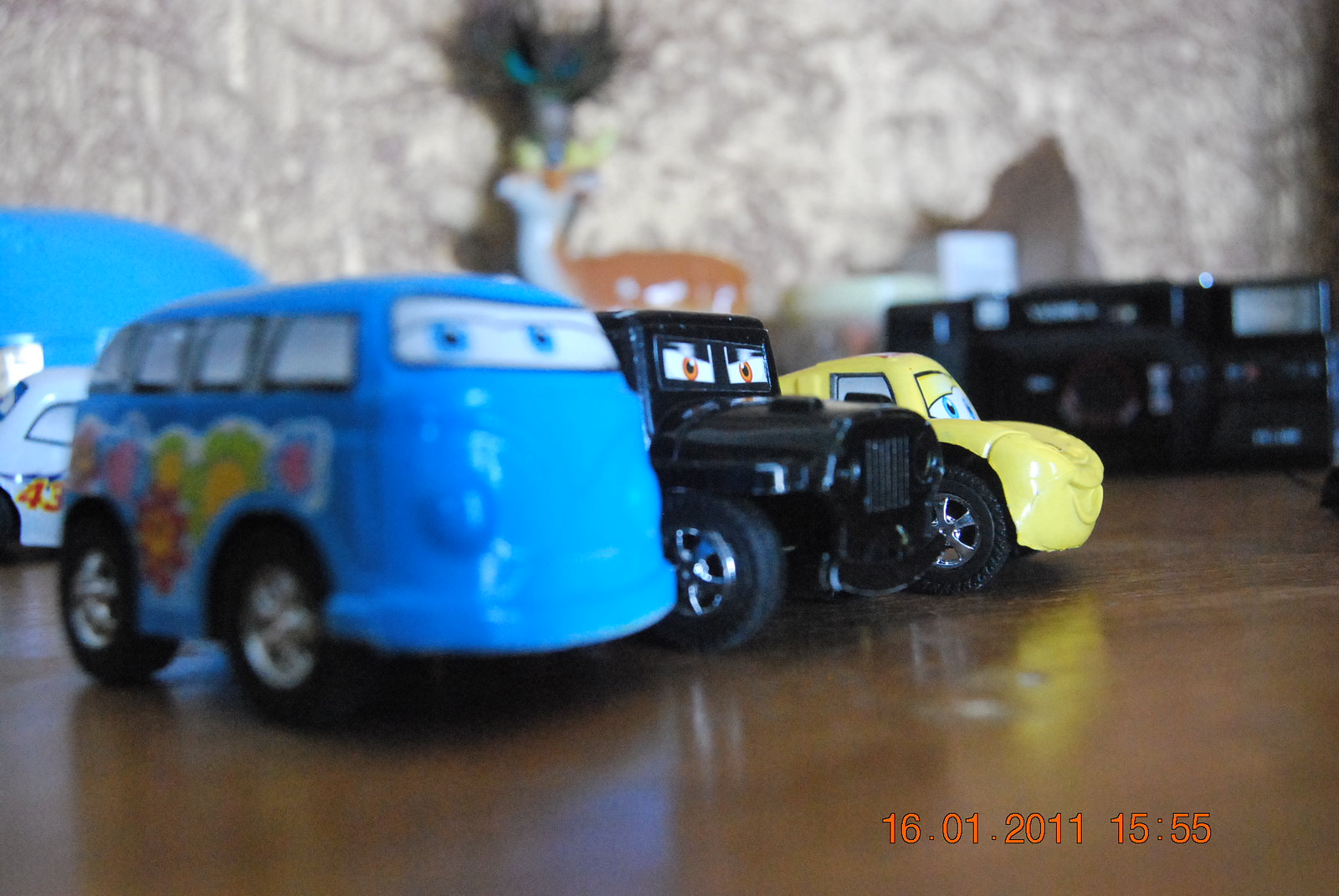The photograph, dated January 16, 2011, at 15:55, captures a light brown wooden surface adorned with various children's toys, prominently from the Disney movie "Cars." Front and center is a blue Volkswagen bus with a whimsical cartoon face, featuring blue eyes with black pupils. It sports multicolored flowers on its side and has black tires with silver rims. To the left of the bus is a black jeep, also with a cartoon face, displaying orange eyes with black pupils and a slightly angry expression. This jeep has black tires with silver hubcaps. Positioned furthest from the viewer is a small yellow Volkswagen Beetle, smiling with blue eyes and equipped with black tires featuring chrome hubcaps. The background features a few other indistinct toy vehicles, blurred against a light tan backdrop, adding depth to the table or desk scene.